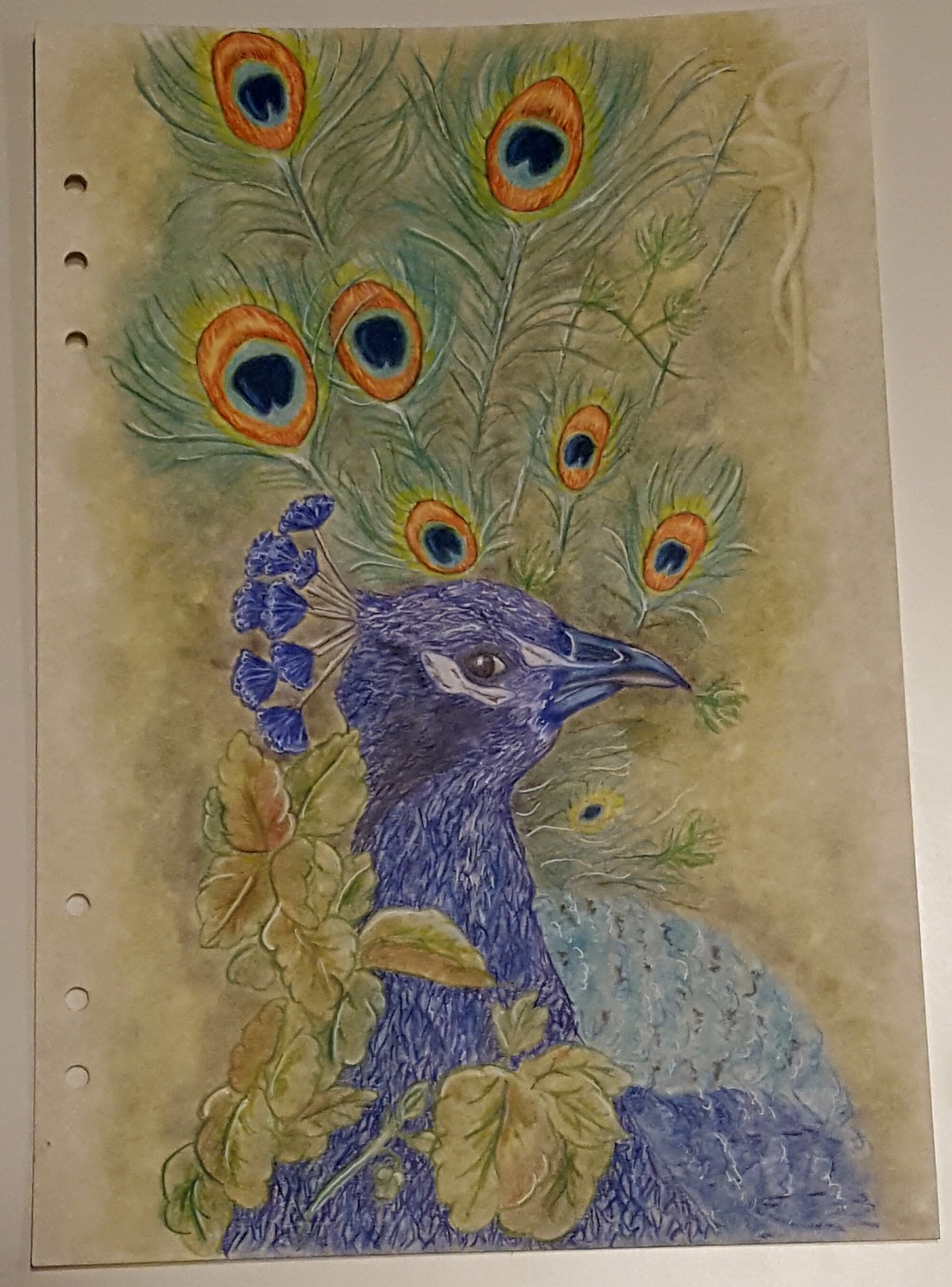This intricate colored pencil sketch features a majestic peacock in a detailed side profile, with its head gracefully turned to the right. The peacock's striking blue plumage dominates the composition, complemented by a matching blue beak and beady black eyes. A distinctive streak of white runs just beneath its eyes. 

The bird's wings are depicted in a lighter shade of blue, adding depth and contrast to its vibrant feathers. Wrapped elegantly around the left side of the peacock's neck are bell-shaped green leaves, enhancing the natural theme of the artwork. The peacock's magnificent tail feathers are primarily green, adorned with intricate orange dots. Each orange dot is intricately detailed with white and black patterns, adding an extra layer of complexity to the piece.

Completing the peacock's regal appearance are blue tassel-like feathers extending from the back of its head. The sketch is meticulously rendered on a sketch pad paper, identifiable by its three punched holes at both the top and bottom left corners. The sketch pad rests on a white table, providing a clean backdrop that emphasizes the vivid colors and fine details of the peacock illustration.